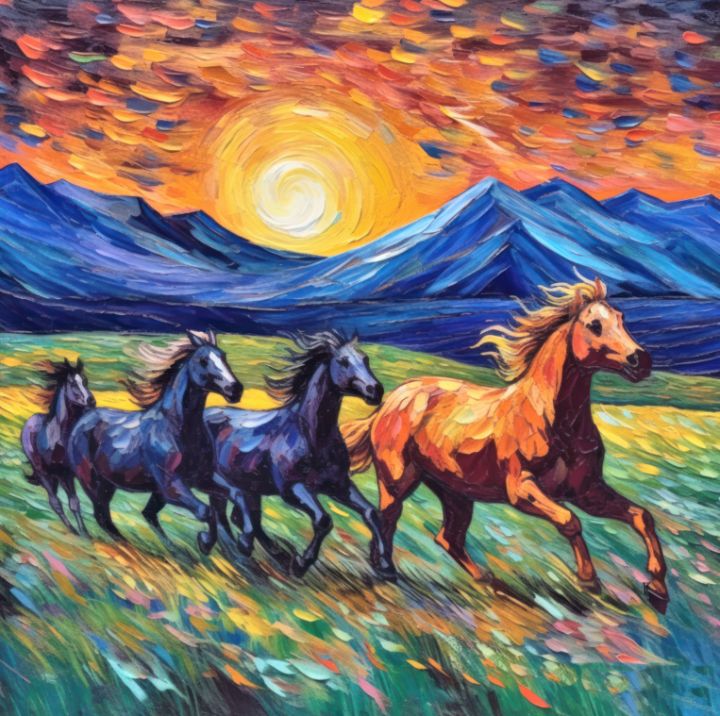This watercolor painting depicts a dynamic scene where four horses gallop through a vibrant field towards the right. The leading horse is painted in rich browns and oranges, while the three following horses are depicted in varying shades of blue and purple. The detailed horses boast flowing manes and some white markings on their faces, adding a touch of realism to their ethereal forms.

The field they traverse is a lush green, accented with hints of yellow, pink, orange, purple, and blue, suggesting an array of wildflowers swaying in the breeze. The brush strokes give the impression of motion, mimicking the wind's effect on the landscape. In the background, blue mountains rise majestically, with subtle touches of tan and brown, creating depth.

Above the mountains, a luminous sun glows at the center of a yellow, swirling sky, flanked by layers of orange, red, and blue hues. The sky becomes darker near the upper left and right edges, adding contrast and drama to the scene. The overall composition captures a vibrant and lively moment in nature, brimming with motion, color, and energy.